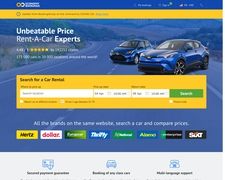The image is a small, square-shaped screenshot of a car rental website. The website features a primarily blue background. Dominating the center, occupying approximately 80% of the image, are two shiny blue cars parked one behind the other, facing left, on what appears to be a deserted desert road. The distant backdrop reveals a desert landscape with small bushes, scrub brush, and patches of grass on the road's left side.

To the left of the cars, there's prominent white text that reads, "Unbeatable Price Rent-A-Car Experts." In the central portion of the image, right beneath the blue cars, sits a long, rectangular-shaped menu with a yellow background. This menu features bold black text that states, "Search for a Car to be Rented," followed by three white rectangular fields for input. Below the input fields, various brand sponsors' logos are visible, including what seems to be the Hertz driving company and Dollar Shave Club. However, the image is somewhat blurry, making it challenging to decipher some of the additional sponsors' logos.